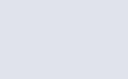A completely blank image featuring a muted, pale gray rectangle. The rectangle is horizontally oriented, being wider than it is tall. The image is devoid of any photographic or illustrative elements, consisting solely of the uniform gray color with no visual content or textual information. There are no people, animals, plants, flowers, trees, buildings, birds, mechanical objects, automobiles, airplanes, helicopters, websites, computers, fish, or food present in the image. It stands as a stark and empty canvas with no additional features or distractions.